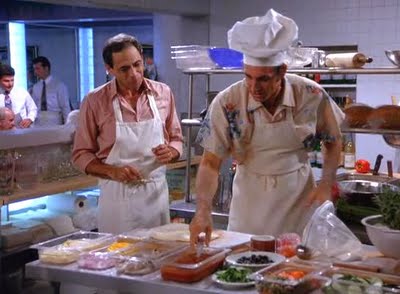In the style of a reminiscent scene from Seinfeld's famed "No Soup For You" episode, this image captures a bustling kitchen environment. Two men stand in front of a prep table laden with an array of Tupperware-like containers filled with diced vegetables. Both are donned in white aprons, immersed in what appears to be preparation for a busy service. The man on the left, with dark hair and a few buttons undone on his pink-peach long-sleeved collared shirt, exudes casual confidence. His counterpart on the right sports a short-sleeved button-up shirt and a chef’s hat nestled behind him, adding to the culinary ambiance. 

The background is filled with kitchen racks, displaying various implements like rolling pins, metal bowls, and additional Tupperware containers. A knife prominently rests near a tomato and a bottle of wine, suggesting the readiness for a sophisticated dish. On the left side, a counter extends towards the back of the room, where patrons — men in white shirts and ties — are seated, possibly engaged in conversation or awaiting their meals. Below this counter, the neatly organized bags, napkins, and butcher paper hint at the meticulous preparation essential in a restaurant setting. High above, though slightly obscured, shelves stocked with glassware complete the comprehensive view of a well-equipped professional kitchen in action.